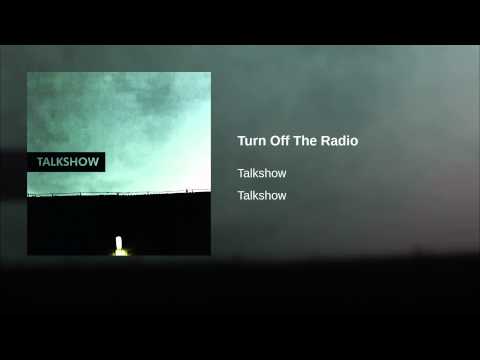The image is a graphic that resembles a music card typically seen on platforms like YouTube or on a car stereo display for audio-only tracks. On the left side of the image, there is the album cover for the band Talk Show. The cover features a striking visual with a greenish, dimly lit sky above a dark, black silhouette, which appears to be either a large wall or a gate with an illuminated door in its center. This creates a somewhat eerie, nighttime ambiance. To the right side of the image, detailed song information appears, all in white text on a gray background. The text reads "Turn Off The Radio" followed by "Talk Show" twice, indicating that the band's name is Talk Show, the album is self-titled "Talk Show," and the song playing is "Turn Off The Radio." The corners of the graphic have a black border, giving the overall image a sleek yet somber look.